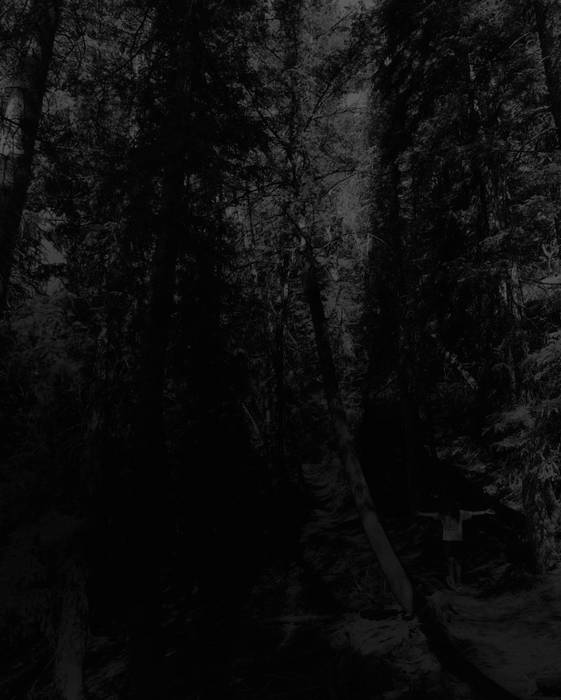The image depicts a somber, dark forest rendered in shades of black, dark gray, and light gray, reminiscent of a pencil drawing. Dominated by trees with an indistinct but fir-like appearance due to the lack of color differentiation, the forest atmosphere is further enhanced by the presence of tree trunks visible in the upper left-hand and center-right sections of the image. The sky has a faintly illuminated spot, possibly indicating the moon. In the bottom right corner stands a figure with long hair, arms outstretched and facing the camera, creating a silhouette effect that makes facial features indistinguishable. The figure appears to embrace the serene but mysterious ambiance of the forest, standing on what resembles a dirt path. The bottom left corner subtly hints at water, adding to the overall mystique and depth of the scene.